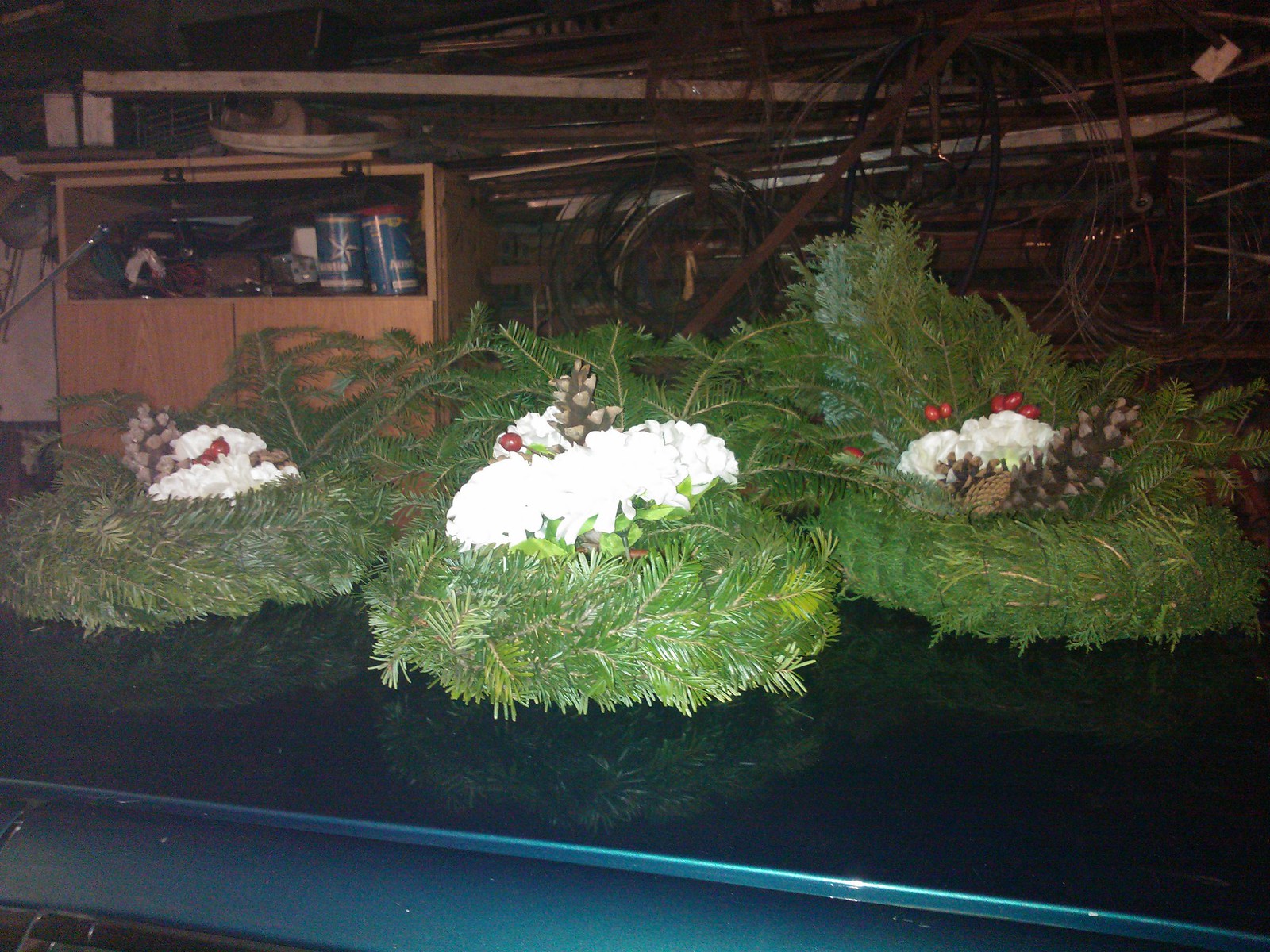In this color photograph, likely taken in a workshop, garage, or basement, a large teal table stands prominently in the center, its shiny surface holding three to six Christmas wreaths. These wreaths, crafted from evergreen or pine-like foliage, feature pinecones, red holly berries, and a white fluffy material that adds a festive touch. To the right of the table, a brown wooden cabinet with an open door reveals an assortment of items, including cylindrical cans – possibly paint – and rolls of wire. The background shows some blue cylindrical objects, which appear to be cleaning supplies. The scene is dimly lit, contributing to a somewhat eerie atmosphere.